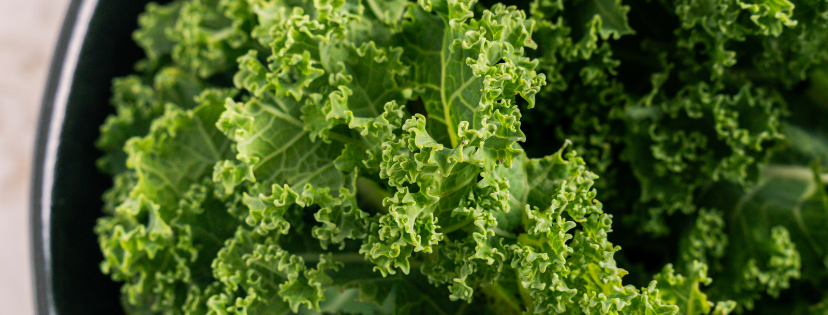This close-up, horizontally-aligned rectangular image showcases a dish filled with deep green, curly leaves, likely belonging to the kale or lettuce family. The bowl, which seems to be either black or dark gray, occupies most of the image, framed on the left edge by a beige countertop or table. The leaves are densely packed towards the middle and left side, where their crinkled texture and thick veins are prominently visible. The right side of the image is less dense, revealing a blurred, lower section of the dish with some empty spots that expose the bowl's dark bottom. The overall texture of the leaves is very curly and frilled, indicative of kale or a similar vegetable.